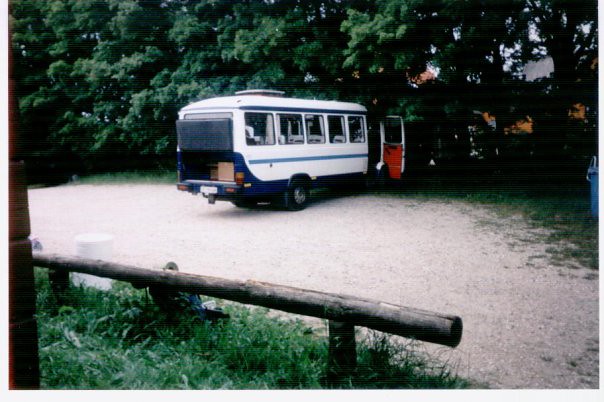This image is an old-style photograph, likely from the 80s or 90s, depicting a small bus parked in an outdoor setting. The bus, which resembles a converted school bus now painted white with a blue stripe, features an open door with a red interior. The bus is situated on a stony, makeshift parking surface that could be a dirt or gravel lot. A small rounded post is positioned near some grass at the edge of the parking area. Surrounding the scene are numerous trees, with glimpses of houses visible through the foliage. There are no people present, but cargo is visible in the back of the bus, suggesting recent activity. The atmosphere suggests the bus may be near an entrance to a park.